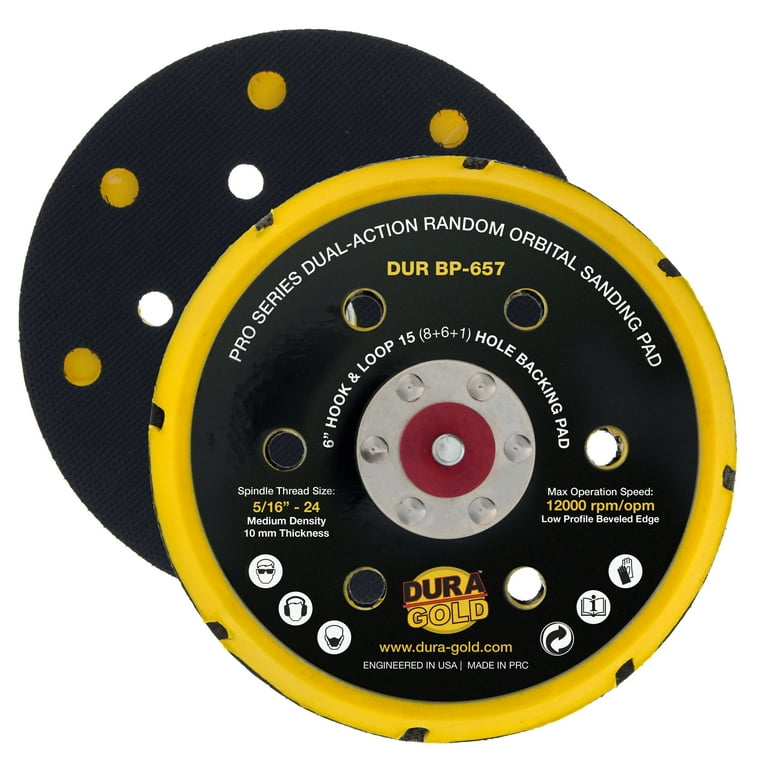The photograph features two circular sanding pads set against a plain white background with no visible borders. Both pads are designed for use with a handheld grinder. The front pad prominently displays the text "Pro Series Dual Action Random Orbital Sanding Pad" around the top edge in white print and is labeled "DUR BP-657" in yellow at the center. Additional specifications, including "6-inch hook and loop 15 / 8 + 6 + 1 hole backing pad," "spindle thread size 5/16-24," and "max operation speed 12,000 RPM/OPM," are printed on the pad.

The pads have a distinctive yellow border and a black center, with the edge lined in red and a small silver metal circle at the very center. The front pad includes several raised, beveled silver circles. Surrounding these labeled details, the pad also features safety pictograms depicting wearing glasses, ear protection, and a face mask. The bottom of the pad showcases the branding "Dura-Gold" along with the website "www.dura-gold.com." It indicates that the pads are "engineered in the USA, made in PRC." 

In the upper left section of the image, part of the second pad is visible, showing several colored holes – two white and four brown – against a black background. Both pads exhibit a low-profile beveled edge with medium density and are 10 millimeters thick.